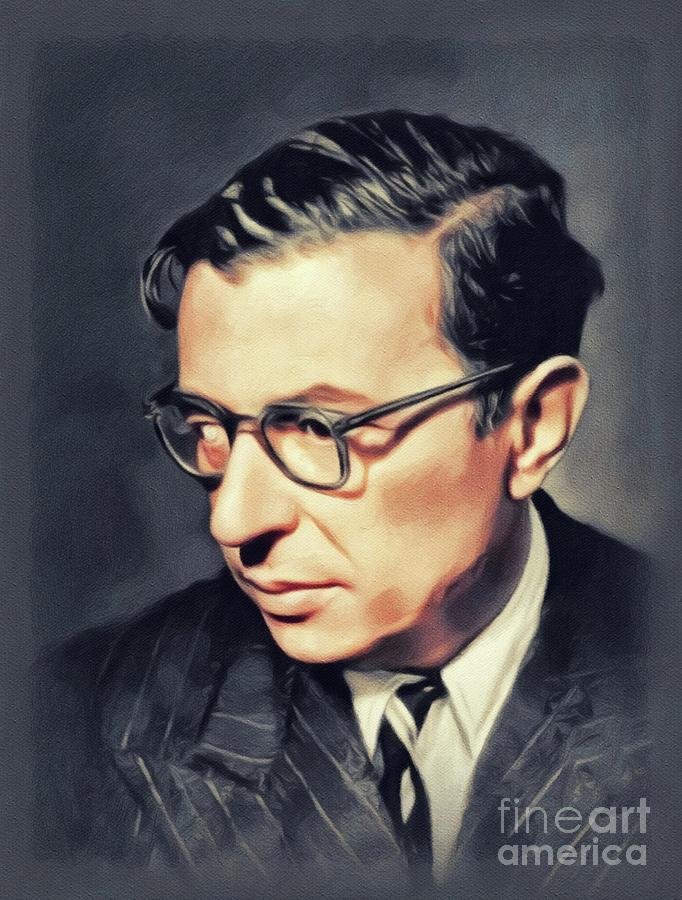The image is a finely saturated, oil painting portrait of a man resembling a 1950s style. The man, who has a beige light skin tone, is depicted wearing gray, thicker plastic-framed glasses, with his right eye appearing lazy and slightly cross-eyed. His black hair, slicked to the right with a touch of gray, complements his brown eyes. He is donned in a gray and white pinstripe suit jacket, a white shirt, and a black and white striped tie. The background features varying shades of gray, from light on the right to dark on the left. The single text in the bottom right corner reads "Fine Art America."